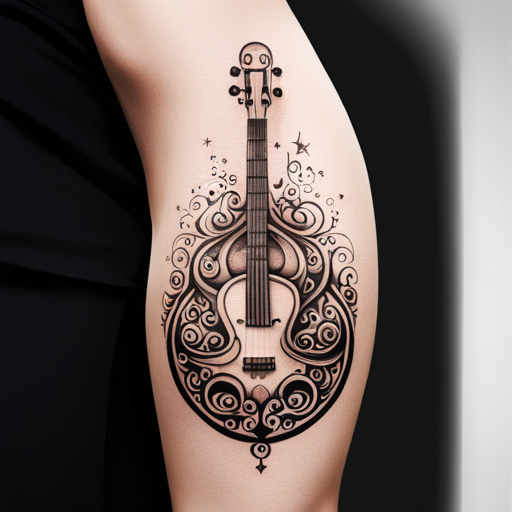This image showcases a detailed tattoo on the inner calf of a person with pale Caucasian skin. The tattoo features an ornate stringed instrument that resembles a lute, guitar, or mandolin, with a large, round body and a slender neck extending upward to a curved end. The design is rich in intricate details, including swirls, floral patterns, and spirals, primarily in shades of black and gray, using the skin tone as part of the background. There are four tuning pegs at the top of the neck. The body of the instrument includes eye-like designs and extensive black shading. Additionally, the tattoo is adorned with decorative elements like bubbles, stars, and possibly a small bird and spade-like patterns. The background of the image is mostly black with a touch of white on the right side. The overall aesthetic is a blend of classical and artistic interpretations, making the tattoo a visually striking piece.